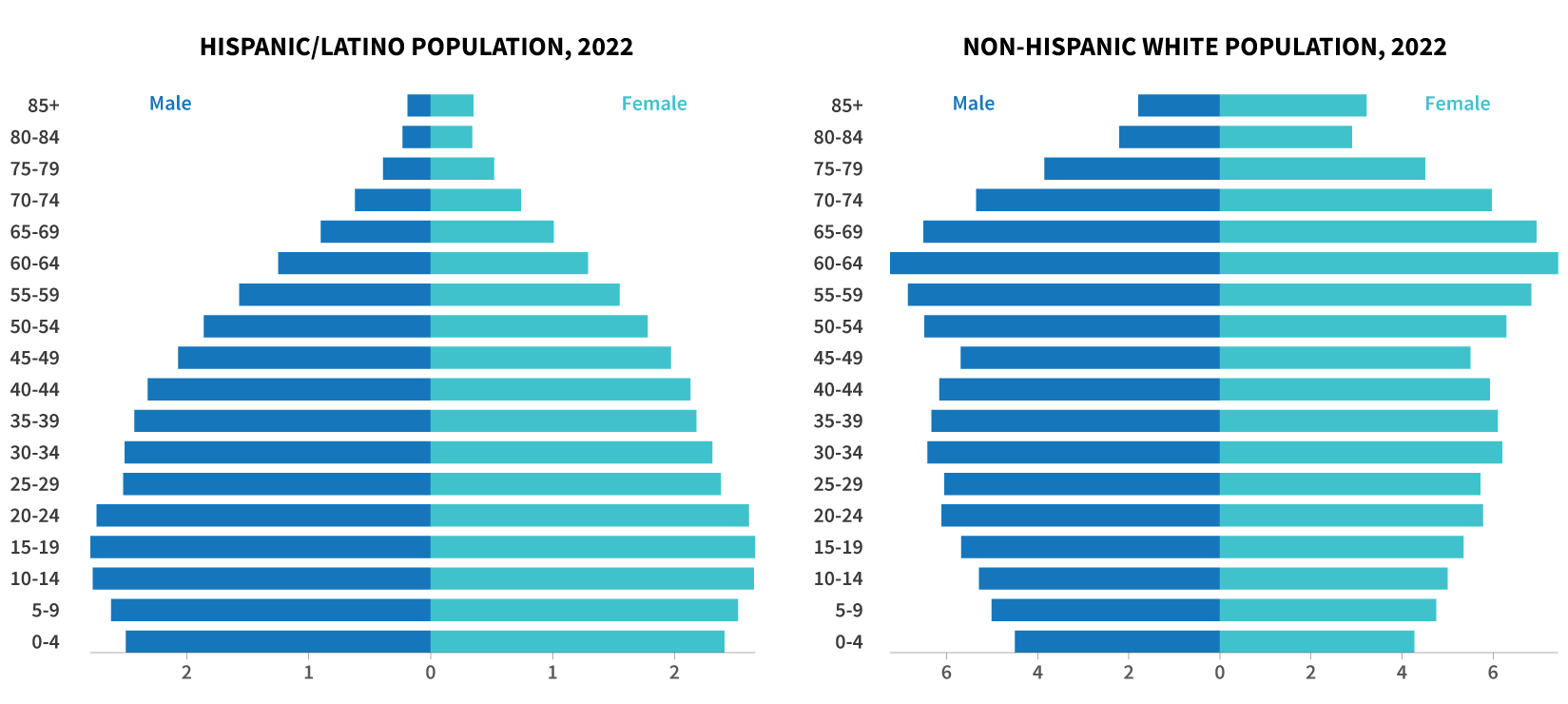The image displays two detailed bar graphs side by side comparing the Hispanic/Latino population in 2022 to the non-Hispanic white population in 2022, segmented by age and gender. The left graph shows the Hispanic/Latino population, while the right graph represents the non-Hispanic white population. Each graph breaks down the data into age groups, ranging from 0-4 years to 85+, with separate bars for males and females. The Hispanic population is notably larger in the younger age groups, particularly from 0-4 through 20-24 years, indicating a significant growth rate among the youth. In contrast, the non-Hispanic white population is more substantial in the older age brackets, specifically from ages 55-59 through 65-69. This striking demographic trend, without specifying a location, suggests a shift in population dynamics, particularly notable for the age groups 15-19 through 45-49 among Hispanics.